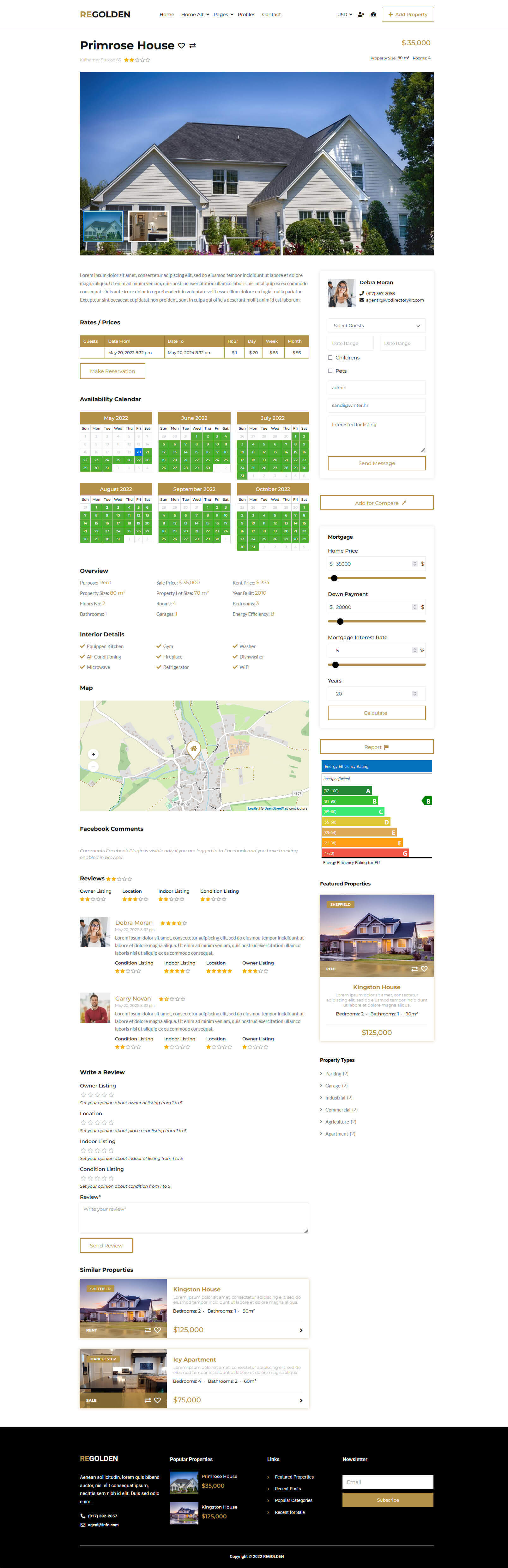The image displays a detailed real estate listing for a property on the "Regoland" website. At the top left, the navigation menu includes options such as Home, Home Wall, Pages, Profiles, Contact, a currency selection for USD, and IMS. The property, identified as "Primrose House," is labeled with a two-star rating. The listed price for the house is $35,000. The property covers an area of 80 square meters and includes four rooms.

In the center of the image, a prominent picture of the house showcases a large residential building surrounded by lush greenery. Scattered around the image are various charts, graphs, reviews, additional pictures, and accompanying text providing detailed information about the property.